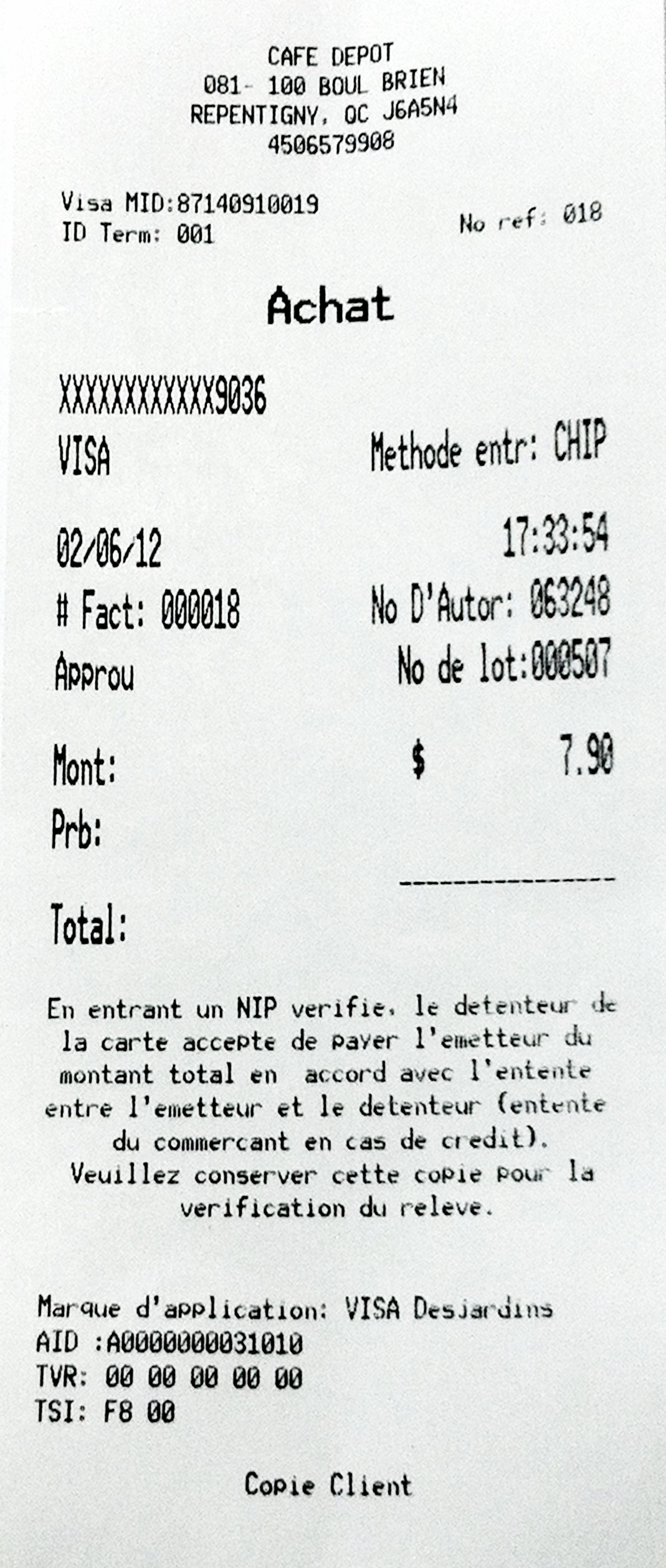This is a photograph of a store receipt from Café Depot, located at 100 Boulevard Brine in Répetini, QC. The receipt is mostly written in French. At the top, the largest text reads "ACHAT," indicating a purchase. Below that, it details transaction information including the terminal ID (001) and a card type identified as Visa, with some numbers partially shown (06020612 and 9036). The purchase amount listed is $7.90. The receipt also includes a date in the format 02-06-2012 and specifies that the payment method was via chip. There is a paragraph in French beneath these details. At the very bottom, it says "COPY CLIENT." The receipt is printed in black text on white paper.